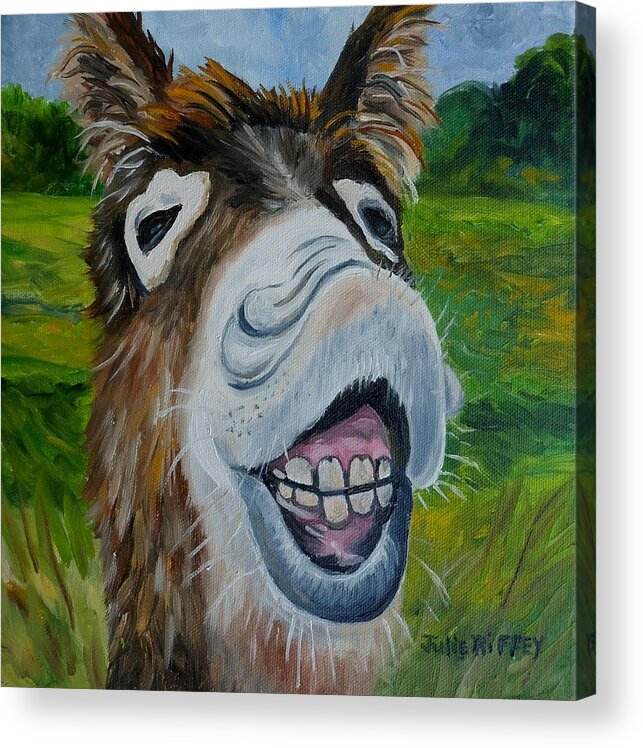The image depicts a vividly colorful painting of a donkey, prominently showcasing only its head. The donkey, which might be mistaken for a llama at first glance, has distinct brown fur, with white patches around its eyes and nose. Its ears are perked up, and its expressive face exhibits a wide-open mouth, showing off its large, goofy teeth and visible gums, giving it a dopey, smiling appearance. The background is a lush, green field dotted with numerous trees, under a bright blue sky, adding to the light and dark contrasts of the painting. The painting is signed at the bottom by the artist, Julie Riffey.